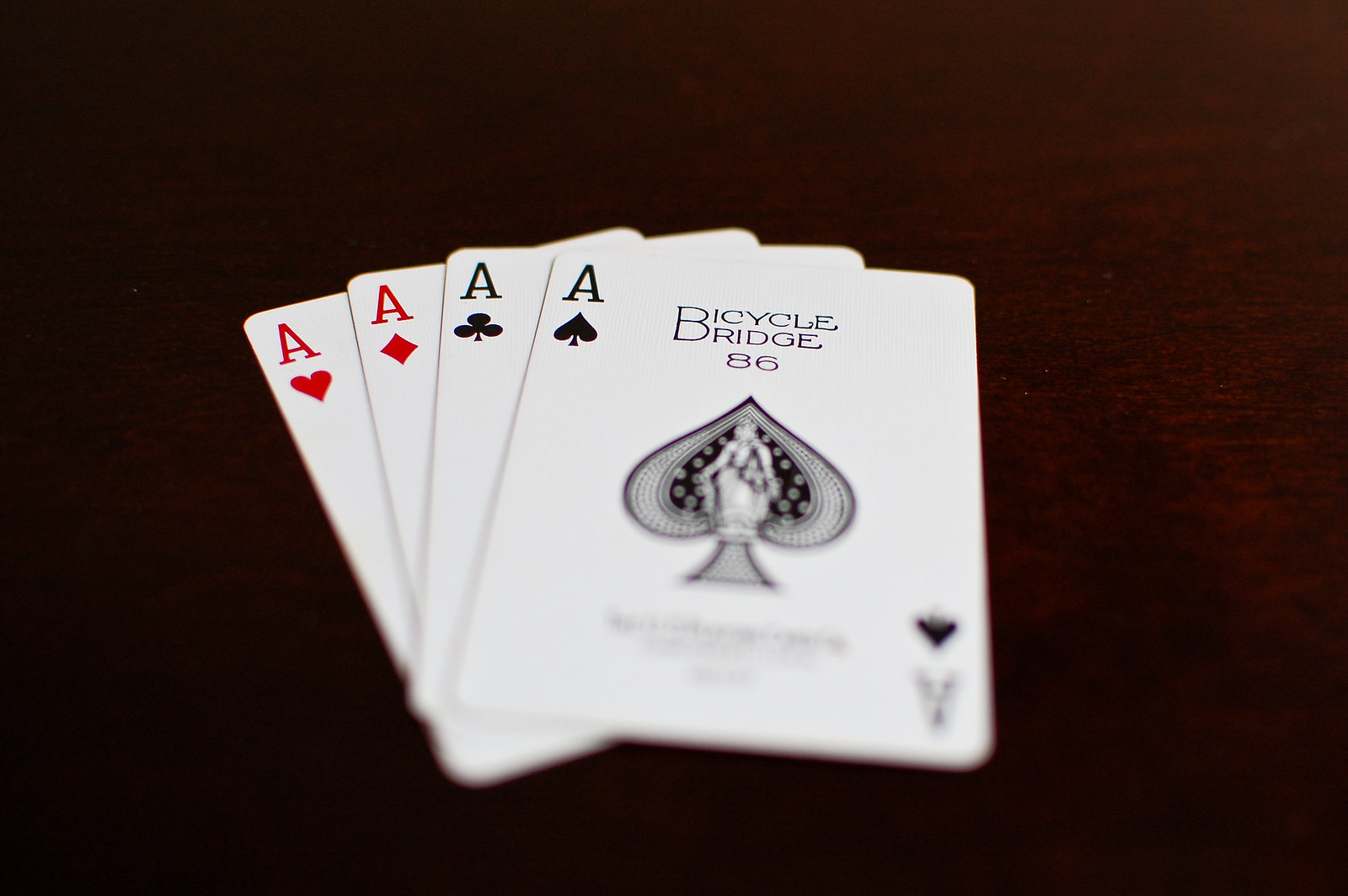This indoor, color close-up photograph captures a meticulous arrangement of all four aces from a deck of cards, fanned out with their lower left corners overlapping. The background is a solid black, adding a dramatic contrast that emphasizes the cards, while the slightly blurry foreground adds a touch of depth.

Starting from the middle of the image, the sequence of aces is as follows: the ace of hearts is at the bottom, followed by the ace of diamonds slightly above and to the right. Next, the ace of clubs is positioned higher and further to the right, with the ace of spades taking the central, prominent position atop the arrangement.

The ace of spades card features distinct black lettering, reading "Bicycle" at the top and "Rider" beneath it, followed by the number 86. Within its iconic spade emblem, there's a partially visible drawing, though it starts to blur. No other words or text are visible in the photograph, and the lower half of the ace of spades is notably blurred.

All the cards appear to be brand new, suggesting meticulous handling and arrangement. The ace of spades is slightly tilted to the right, adding a subtle dynamic to the composition. The cards are seemingly set on a dark wooden table, though this detail is not entirely clear due to the photograph's framing and focus. No other objects or elements are present in the image, keeping the viewer's attention squarely on the elegant display of the four aces.